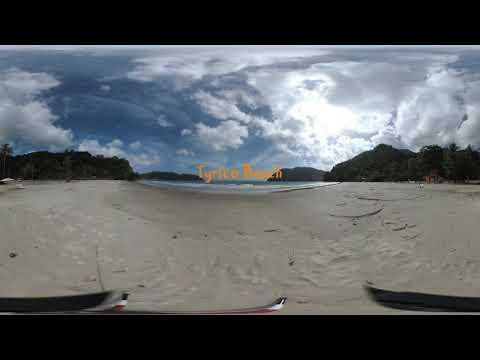The image captures a beach scene, identifiable by the text "T-Y-R-I-T-O Beach" in the center. The photograph appears to be taken with a fisheye lens, which creates a distorted, panoramic view. The foreground is dominated by a smooth, sandy shore that has a grayish, clay-like texture and lacks vegetation or rocks. The shoreline meets a strip of blue water, hinting it is either an ocean or a lake. Surrounding the water on both the left and right sides, there are clusters of densely packed green trees, forming a natural border. The sky above is vibrant with a mix of fluffy white and gray clouds, partially covering the sun, but allowing patches of blue sky to peek through. The overall scene has a serene and expansive feel, combining the elements of sand, water, trees, and a partly cloudy sky.